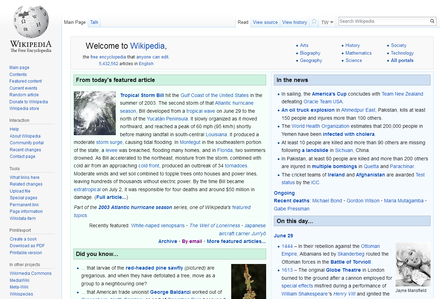The image depicts a Wikipedia page, featuring a cluttered and somewhat difficult-to-read interface. At the top, it prominently displays "Welcome to Wikipedia" in a large font. The left-hand side showcases a gray sidebar adorned with a globe icon and several blue hyperlinks, none of which are legible in this context. Directly right of the sidebar, another header echoes "Welcome to Wikipedia," alongside a gray bar with blue text beneath it.

Positioned below this section, there's a highlighted portion titled "From Today's Featured Article," which discusses a tropical storm, though its name remains unreadable. This segment is distinguished by a green background with black and blue text. Above this article, you can see navigation links like "Main Page" and "Talk," with additional options beyond visibility. On the page's upper right, there's a Wikipedia search bar.

Further down, a bar reads "Did You Know?" and is followed by intriguing facts in blue text. To the right, a section with a blue background and a prominent blue bar titled "In the News" stands out, featuring bolded black text and various bullet-pointed updates in black and blue text. The final segment, labeled "On This Day," notes historical events that occurred on June 29th, presented through several bullet-pointed entries.